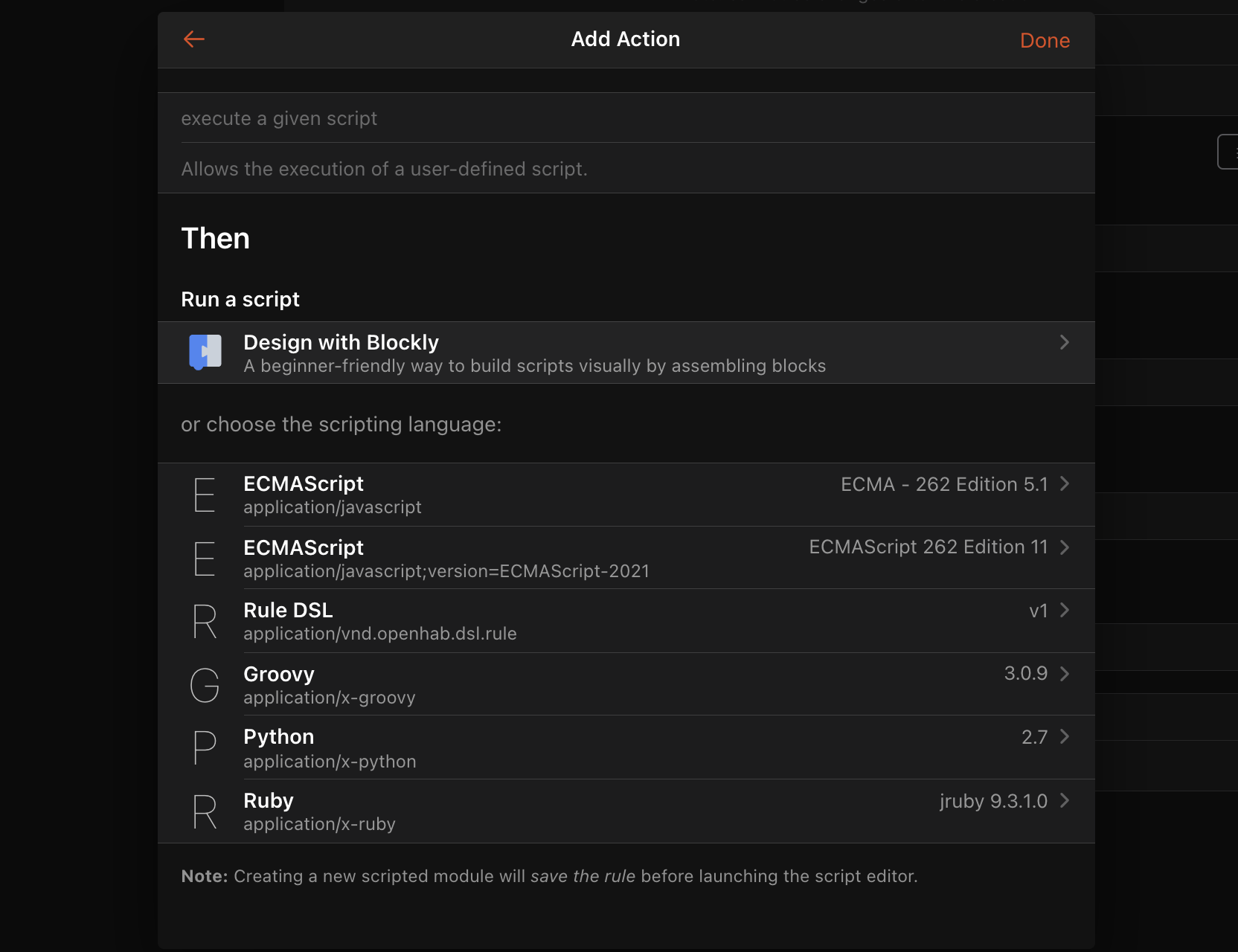The image serves as a guide for users looking to add action to a specific interface, particularly involving scripts. It features a predominantly black background with a few accent colors—white for most text and red for some key elements.

In the upper left corner, a red arrow points to the left side. Centered at the top, the phrase "Add Action" is displayed in white, while the word "Done" appears in red on the right.

The main body of the image introduces several script-related instructions. The first line reads, "Execute given script," explaining that this option allows the execution of a user-defined script. Below this, the word "Then" is written in white, followed by the phrase "Run a script."

Further down, the term "Design with Blockly" is highlighted, noting that it’s a beginner-friendly method to construct scripts visually by assembling blocks. Accompanying this note is a small, blue-and-white halved square icon.

At the bottom, there is an option to choose the scripting language. An adjacent dropdown menu lists the following in capital letters: "E, E, R, G, P, R." These abbreviations stand for various scripting languages:

- E: ECMA Script
- R: Rule DSL
- G: Groovy
- P: Python
- R: Ruby

Additionally, there is a note stating that creating a new scripting module will save the rule before launching the script editor.